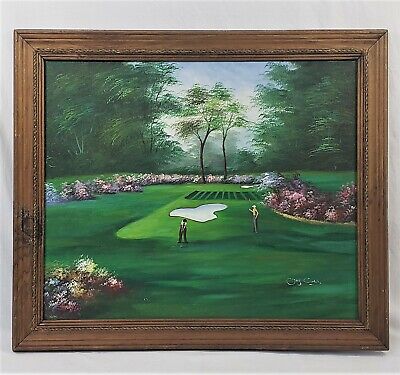The image is an oil painting hung on a white wall, framed within a rather thick, medium-colored wooden frame embellished with decorative curves and etching, giving it an aged appearance. The painting captures a serene golf course scene with a muted color palette. Dominating the foreground, a putting green is depicted with two men engaged in the game; one is bent over, preparing to hit a golf ball, while the other holds the flag, standing near a sand trap. Encircling the putting green is a colorful flower bed with hues of pink and white, bordered by manicured cement edges. In the background, tall deciduous trees and lush forests stretch across the scene under a clear blue sky, adding depth and tranquility to the picturesque golf course setting.